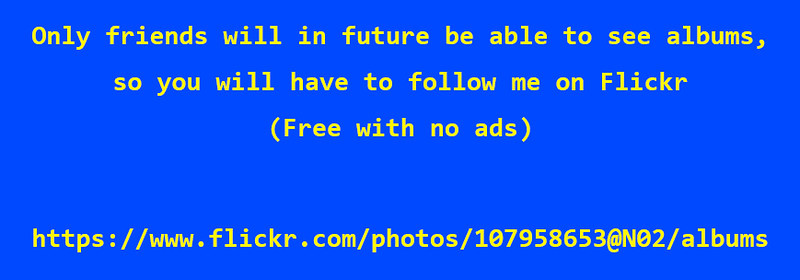The image is a computerized snapshot featuring a blue rectangular background with prominently displayed yellow text. The text is spread across four lines, primarily at the top and one at the bottom. The message reads: "Only friends will in future be able to see albums, so you will have to follow me on Flickr (free with no ads)." At the bottom of the image, the website address is located: "https://www.flickr.com/photos/107958653@n02/albums". The image does not contain any people and focuses solely on conveying the informational text.